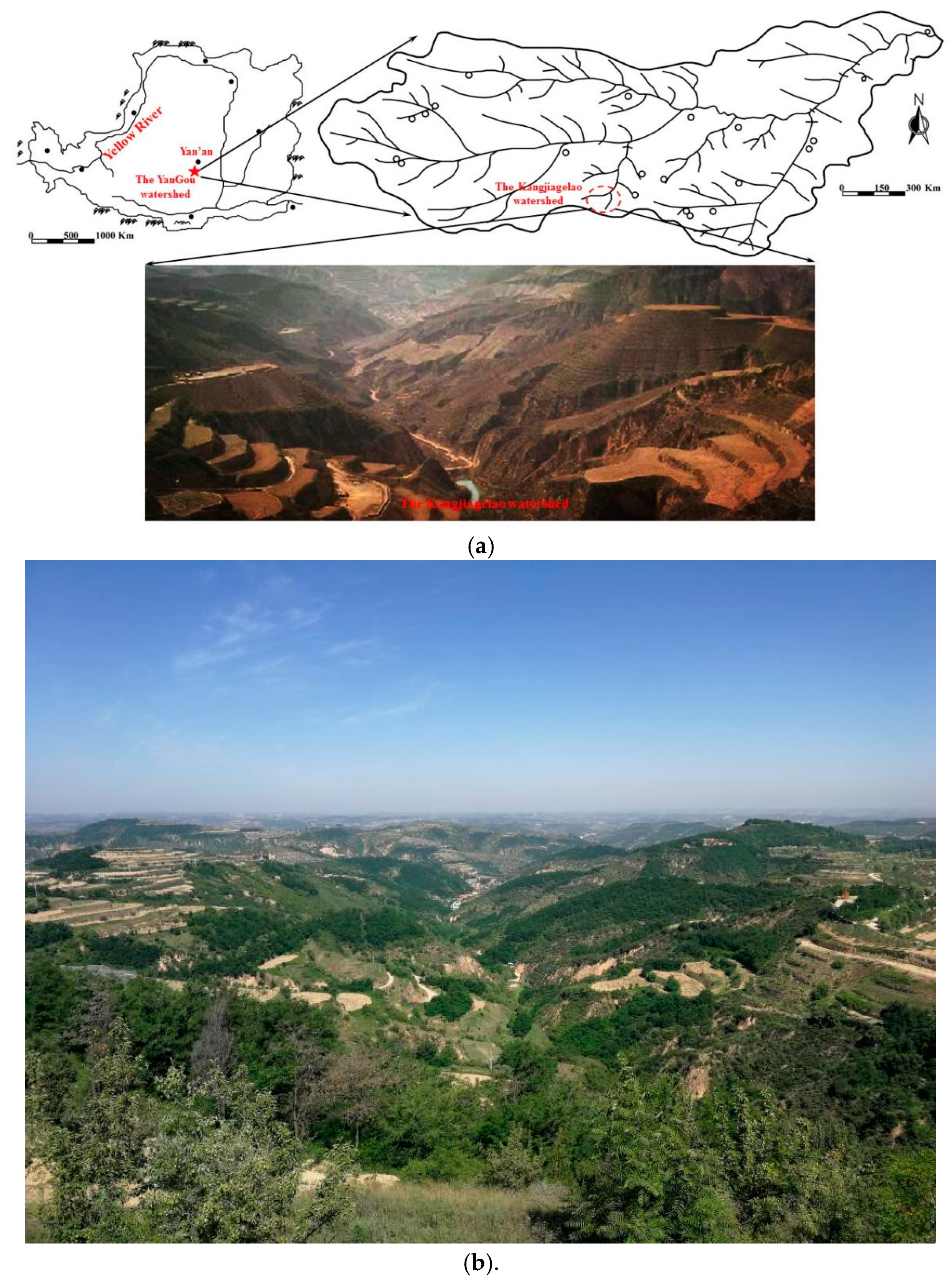This image, designed as an educational visual aid in portrait orientation, presents two horizontally oriented, rectangular photos displaying a transformative environmental scene. The top part of the aid includes a detailed black-and-white map highlighting regions like the Yellow River, Yan'an, and the Yangou Watershed, with various watershed areas marked prominently in red. The first photo labeled "A" captures a deep, brown, rocky canyon area, characterized by irregular, mined-out valley sides, emphasizing the rugged and harsh terrain of the region. Below it, the second photo labeled "B" showcases a dramatic change—a lush, green, and hilly landscape, indicating the area has been replanted and revitalized. The clear blue sky with clouds hints at a typical daytime setting, with a notable haze in the distance. The transformation from a barren canyon to a regenerated, green terrain is effectively illustrated, highlighting both geological features and ecological restoration efforts.